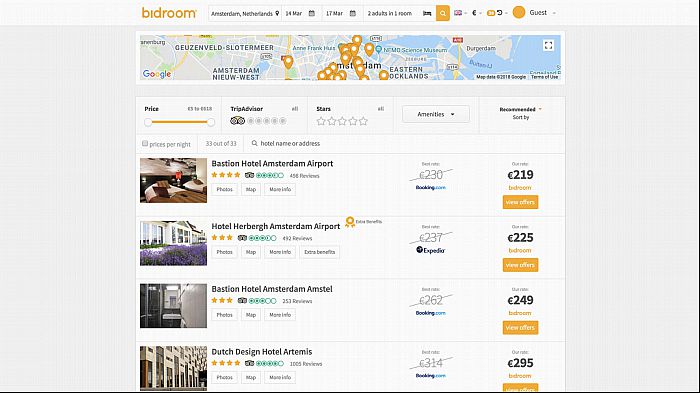Screenshot of a search results page for hotels in Amsterdam, Netherlands, hosted by Bidroom. The top left corner features the Bidroom logo in mustard-colored lowercase font, alongside the search bar for the destination. Next to it, there are two calendar bars for selecting dates, currently set from March 14 to March 17. Adjacent to these is a bar for specifying the number of adults and rooms, followed by various icons.

Below this interface is a slim map of Amsterdam, dotted with mustard-colored markers indicating hotel locations. Concentrated clusters of these markers are visible in the central area of the city.

Further down, the page displays an array of filters. Users can slide a bar to set the price range, select hotel star ratings from one to five, choose desired amenities from a drop-down box, and apply additional filters.

The search results themselves are listed below these options. Each result includes a photograph of the accommodation, its name, star rating, price per night, and a “View Offers” button in mustard-colored font. Four distinct hotel options are visible in this screenshot.